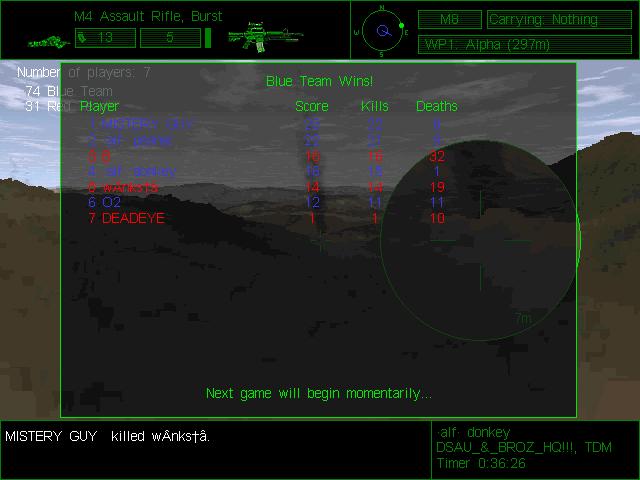The image appears to be a screenshot from a video game, likely a first-person shooter, showcasing a post-game summary. The background features a dark, brown and gray mountain terrain with dim lighting. Superimposed over this backdrop is a semi-solid, semi-transparent black box with a green border. Inside the box, in green text, it prominently displays "BLUE TEAM WINS" at the top. Beneath this, there are multiple columns listing player names on the left, and their respective scores, kills, and deaths to the right. At the bottom of this box, it states, "Next game will begin momentarily," also in green.

Additionally, various game statistics and messages are dispersed throughout the screen. At the very bottom, a chat message in white text indicates, "mystery guy killed WANKSTA." The top of the screen has diagrams of two guns, with annotations such as "M4 Assault Rifle Burst 13" and "MB carrying nothing WP1 Alpha 297M" in green text. A timer reads "03626," and player aliases like "ALF donkey" are mentioned on the right-hand side. This amalgamation of details provides a comprehensive look into the end-of-game interface for the depicted video game.